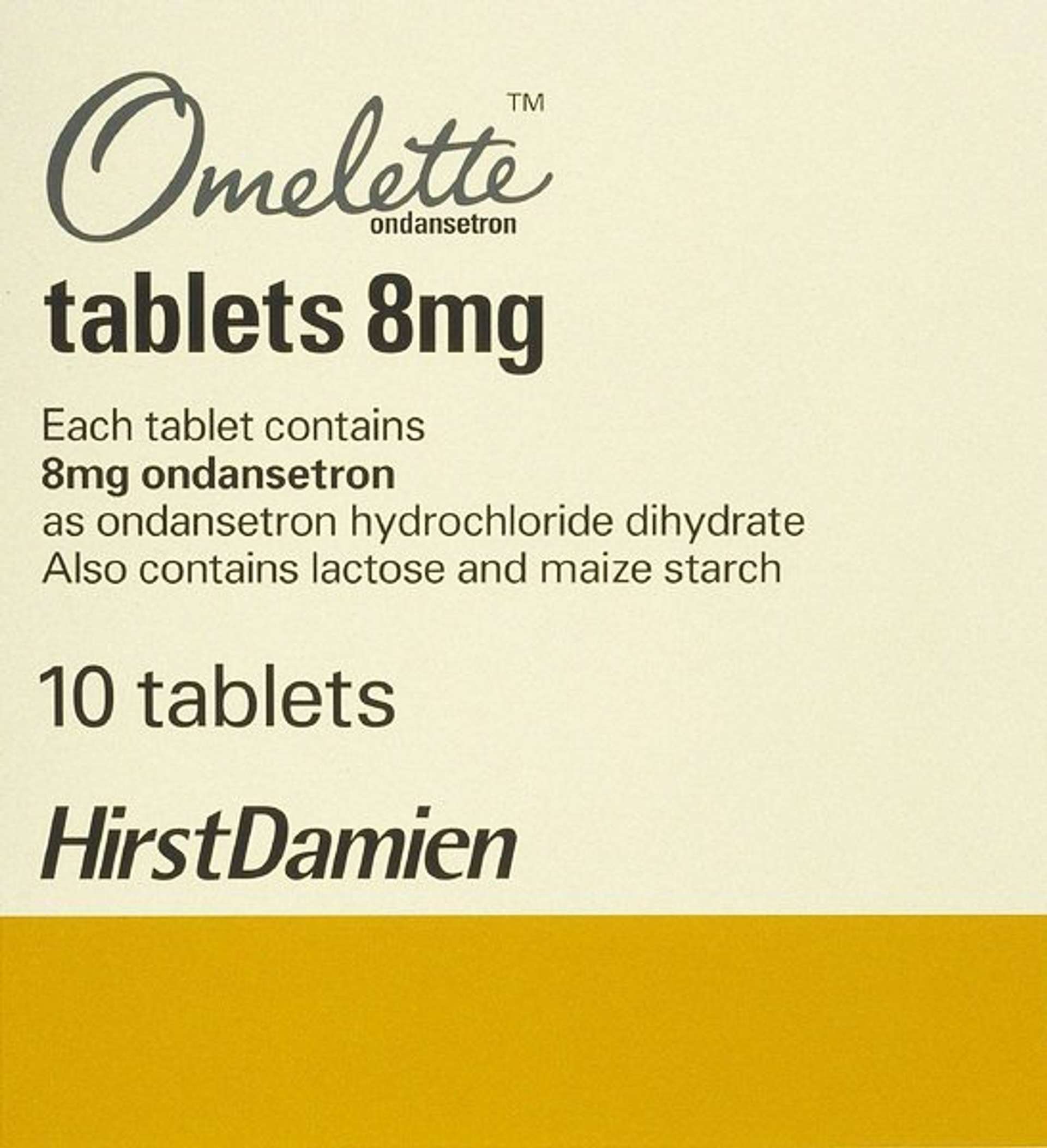The image depicts a pharmaceutical drug box with a cream-colored background. At the top, the trademark "omelette" is written in cursive script. Directly below, andanestron is noted, with additional specifications stating the contents as "ondansetron tablets, 8 mg." The text explains that each tablet contains 8 milligrams of ondansetron, specifically as ondansetron hydrochloride dihydrate. It also mentions that the tablets contain lactose and maize starch. The box contains 10 tablets, and the name "Hurst Damien" is prominently displayed at the bottom of the packaging. Across the bottom of the box, there is a distinctive mustard yellow band.